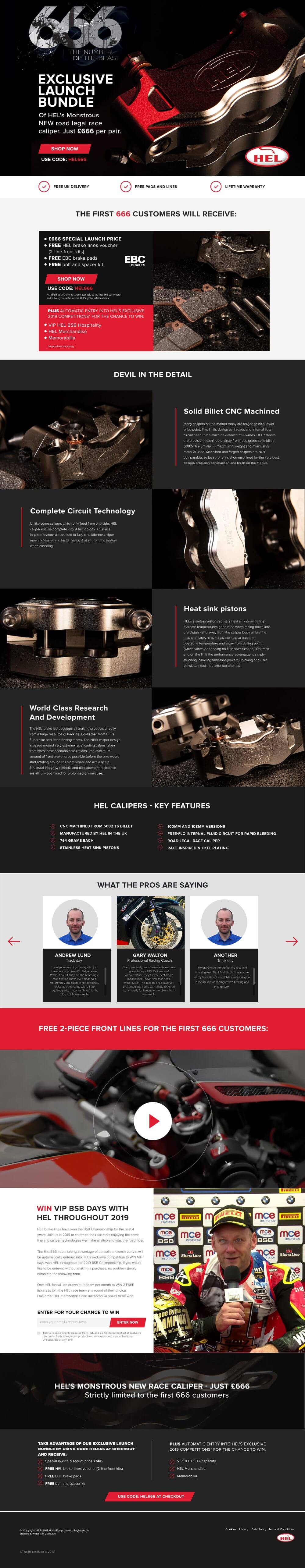The image depicts a section of a website with a racing theme. Prominently displayed at the bottom of the image is a well-dressed man, identified as a white gentleman, who is wearing a sleek racing suit adorned with multiple patches. He is holding a microphone to his mouth and also dons a hat, reinforcing the impression of a professional motorsport setting. The suit he is wearing resembles those used in high-performance racing, such as Formula 1.

To the left of this individual, there is a play button which is presumably linked to a video. Accompanying the play button, there appears to be the image of a motorcycle, suggesting that the website might cater to both car and motorcycle racing enthusiasts.

The overall color scheme of the page is dominated by black, white, and red. Near the top of the image, the text "Exclusive Launch Bundle" is prominently displayed along with the number "666" and the letters "HCL", potentially indicating a promotional offer or product bundle from a specific brand. Additionally, there are several images of men and another play button, hinting at more multimedia content available on the page. The black and white background with red accents frames the content, creating a striking visual appeal that aligns with the high-energy world of motorsports.